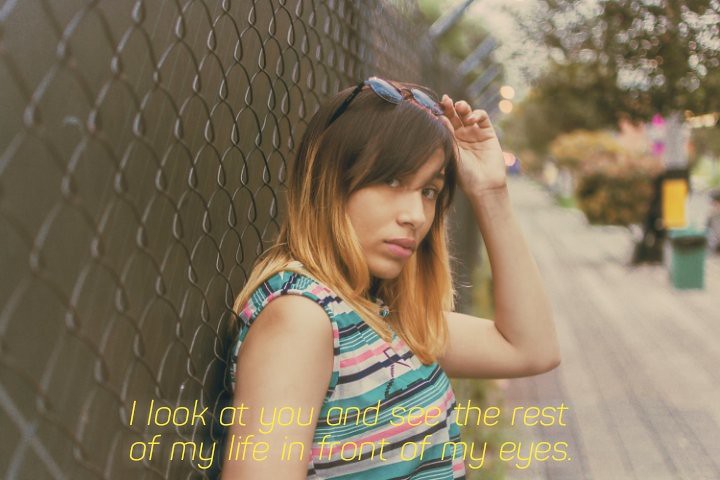This vibrant summertime photograph captures an intriguing scene of a woman standing against a chain link fence. Her ombre hair transitions from dark brown at the roots to blonde towards the ends, framing her face with shoulder-length waves. She is dressed in a colorful, horizontally striped tank top, featuring shades of white, turquoise, navy blue, and pink. The woman strikes a captivating pose, with her left hand pulling back a pair of sunglasses through her hair. Her head is turned left, while she gives a side-eyed, intense gaze towards the camera. The background, blurred and out of focus, reveals a street, some foliage, trees, and possibly a trash can, contributing to a sense of summertime leisure. Text in yellow letters overlays the image, reading, "I look at you and see the rest of my life in front of my eyes," with a subtle blur effect added behind the text for emphasis.